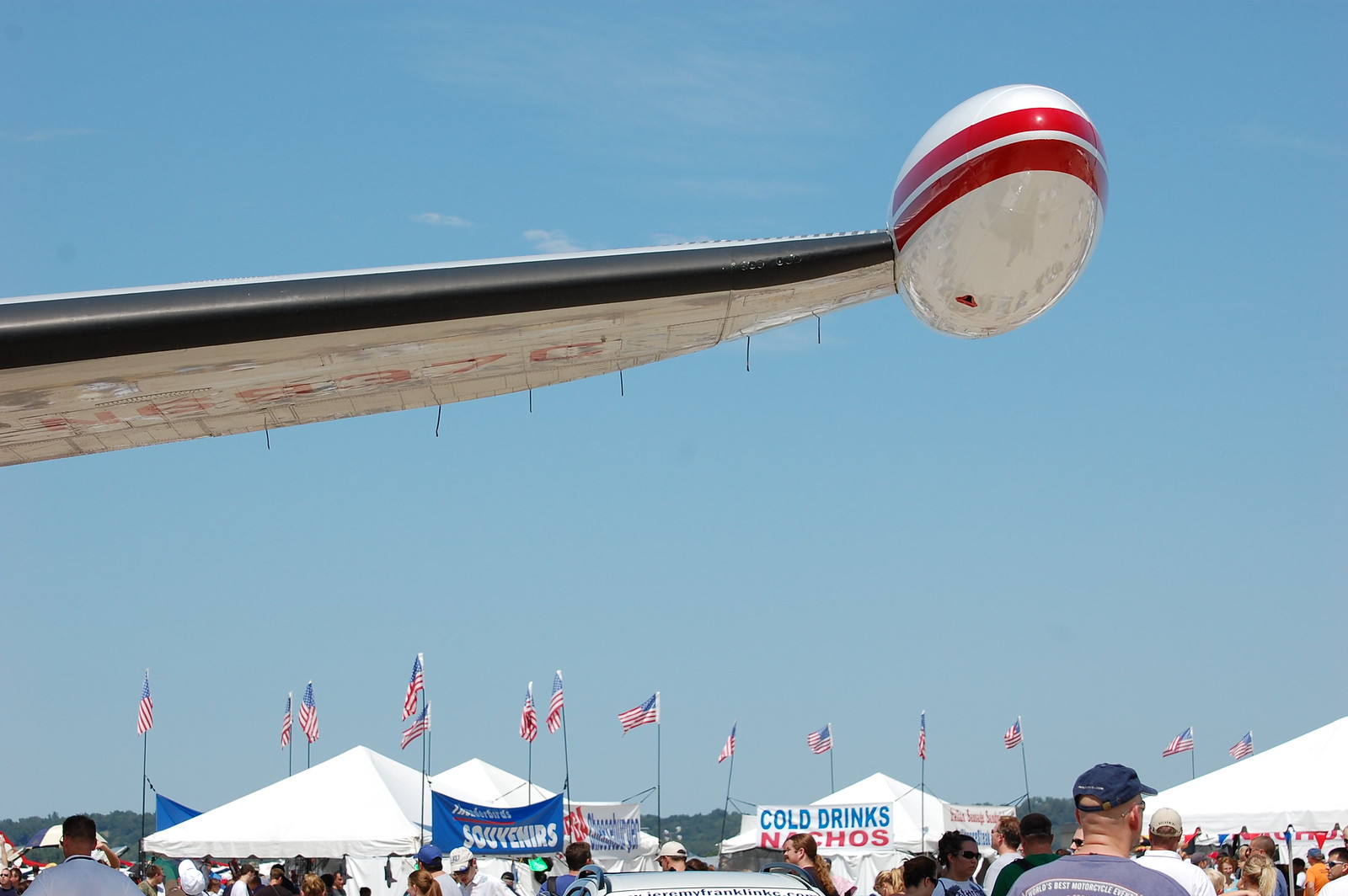This wide, rectangular image captures the bustling scene of an air show. Dominating the top half of the picture is the wing of an airplane, which extends from the middle left of the image and tilts slightly upward diagonally. The wing, crafted from a dirty white material, features a black stripe running along its edge, culminating in a white, oval-shaped object adorned with two red stripes. The backdrop of the sky is mostly blue with a few tiny white clouds scattered throughout.

In the bottom half of the image, several white triangular canopy tents are visible, each adorned with multiple American flags at the corners. The tents are a hive of activity, with numerous heads and shoulders of people milling about. Among the various tents, one prominently displays a white sign with “cold drinks” in blue text and “nachos” in red. Another sign advertising souvenirs is also visible. A notable detail includes a man wearing a baseball cap in the bottom right corner of the image. The scene vividly conveys the lively atmosphere of the event, set against the striking backdrop of the airplane wing and the open sky.